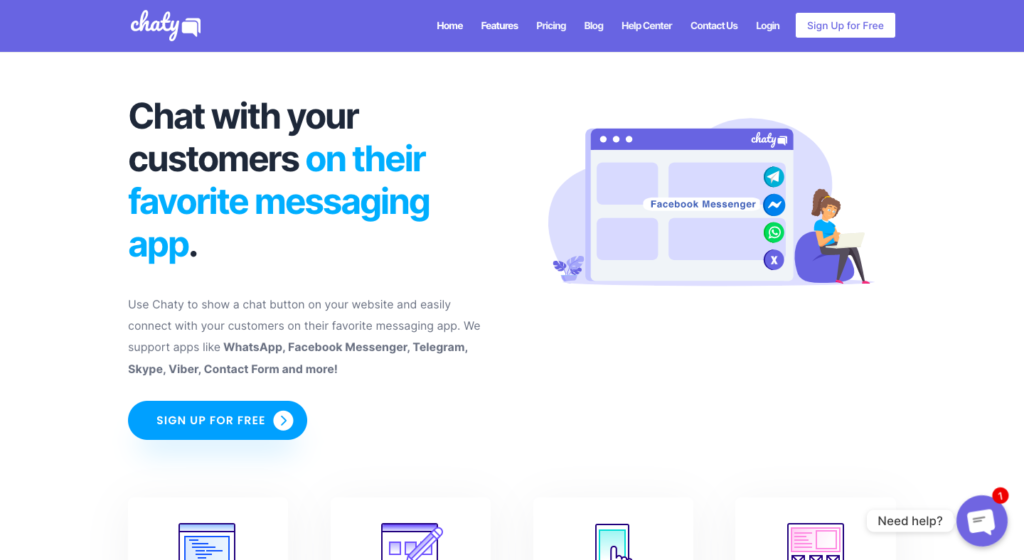A website features a top navigation bar with a long purple strip. On the left side of the strip, the word "CHATY" is written in cursive, accompanied by a white speech bubble icon to its right. The navigation options listed from left to right are: Home, Features, Pricing, Blog, Help Center, Contact Us, and Login. There is also a white rectangular button on the far right with the text "Sign Up for free." 

Beneath this navigation bar, the title "Chat with your customers" is displayed in black text, followed by a blue subtitle: "on their favorite messaging app." Additional explanatory text reads: "Use CHATY to show a chat button on your website and easily connect with your customers on their favorite messaging app. We support apps like WhatsApp, Facebook Messenger, Telegram, Skype, Viber, Contact Form, and more." A blue circular button below this text also reads "Sign Up for free."

To the right of this introductory text, there is an image of a woman sitting in a purple beanbag chair. She wears a blue shirt and black pants, with her brown hair tied in a high ponytail. A laptop rests on her lap. In the lower right corner, a help prompt reads "Need Help?" next to a purple circle with a white chat box icon that has a small red notification bubble labeled with the number one.